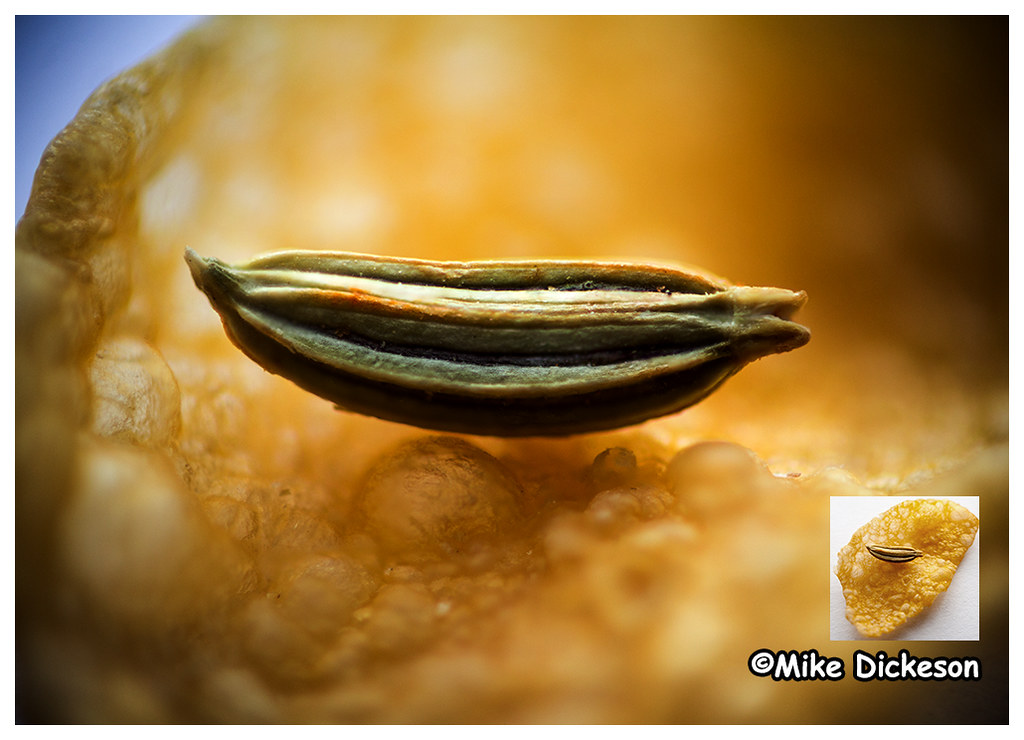This image is a highly detailed, close-up view primarily filled with shades of yellow, interspersed with white and darker, almost brown hues. Dominating the scene is a textured object, resembling a cornflake or a thick potato chip, puffed up with bubbles and intricate details. Near the center of this yellow mass rests a small, elongated, green seed with noticeable ridges running along its length, somewhat banana-shaped. In the bottom right corner, there’s a white square inset showing a more zoomed-out depiction of the same yellow textured object and seed, providing context to the main image. A blue background occupies the upper left corner, transitioning to black towards the right. Beneath the white square inset, the photographer’s name, "Mike Dickinson," is prominently displayed.